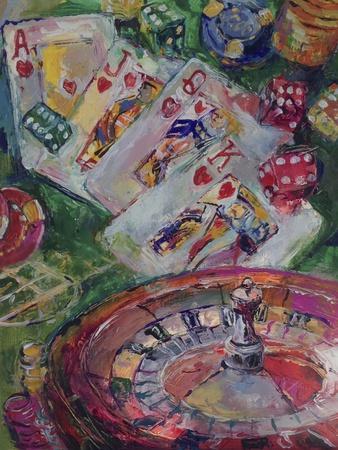The image depicts a vibrant, watercolor painting reminiscent of a casino scene. At the center, four playing cards—Ace, Jack, Queen, and King of hearts—are arranged from the upper left to the middle right, characteristic of a Royal Flush. Due to the watercolor medium, the details on the face cards are somewhat blurred, lending a soft artistic touch to the depiction. Above the face cards, two red dice are placed over the Queen and King, and a green die can be seen above the Jack as well as another between the Ace and Jack. A yellow die subtly peeks out between the red ones.

In the upper right corner, there are piles of chips, primarily yellow and blue, though the blue appears to be a single chip while the yellow is a stack. In the lower half of the image, a roulette wheel stretches from the bottom right to nearly the bottom left, characterized by red and variously colored circles, with a long handle-like extension emanating from its center. Interspersed throughout the scene are additional stacks of chips, adding to the lively casino atmosphere, all laid out on what appears to be a green felt table background.